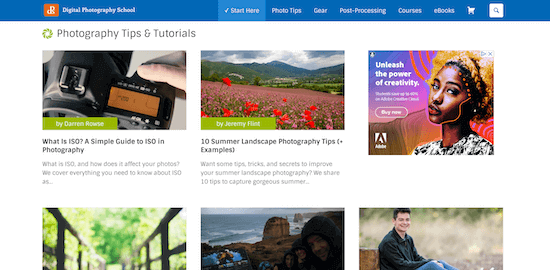This webpage features a clean white backdrop with a prominent blue navigation bar across the top. On the left side of this bar is an orange box displaying a white logo comprised of a white line looping around in a distinctive pattern. Adjacent to this logo, in bold white text, are the words "Digital Photography School." Centrally located within the blue bar are several clickable tabs for easy navigation. The first tab, highlighted in a lighter shade of blue, bears a checkmark and reads "Start Here," indicating it has been selected. Following this are tabs labeled "Photo Tips," "Gear," "Post-Processing," "Courses," and "E-books," the latter accompanied by a white shopping cart icon. A white box containing a blue magnifying glass icon serves as a search feature on the far right.

Below the navigation bar, the page displays a grid of images arranged in two rows of three. 

- The first image is of a sleek black camera held by a hand entering from the right side, with the caption, "What is ISO? A Simple Guide to ISO in Photography," in black text beneath it.
- Next to this, a vibrant photograph captures a field of red and pink flowers, grassy fields, distant hills, mountains, and a blue sky. The caption reads, "10 Summer Landscape Photography Tips (+ Examples)."
- The third image in this row features an AI-generated likeness of a black woman with blondish afro curly hair, dressed in a white and black T-shirt.

The second row includes:

- An image that appears to be taken from a low angle, focusing on a bridge with brown rails.
- Next to this is a photograph of several individuals in black rain jackets with their hoods up, standing against a backdrop of brown rocks and a gray sea. Four people are clearly visible, though the row extends beyond the picture's frame.
- The final image shows a Caucasian boy with short dark hair, seated with his back to a brown tree stump. He wears a black zip-up shirt with a collar and blue jeans, facing away from the left side of the picture.

This meticulous layout and color scheme emphasize the structured and user-friendly nature of the Digital Photography School website, catering to photography enthusiasts with various educational resources.